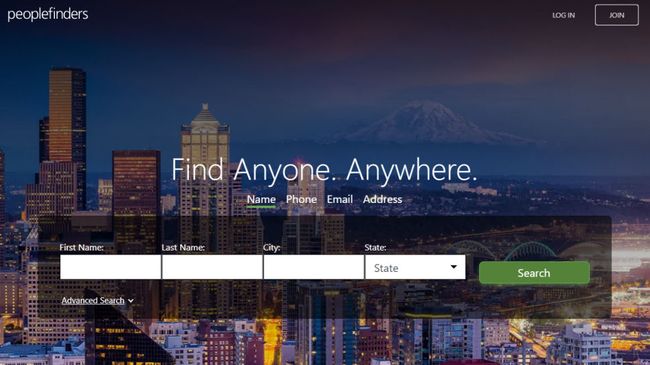The screenshot captures a vibrant evening city skyline, illuminated by numerous lights in the buildings against a partly foggy backdrop. In the foreground, a web interface for a people search tool is displayed prominently. The tool features fields for entering details such as first name, last name, city, state—where the state box is notably highlighted—and advanced search options. A green rectangle with the word "Search" in white text is easily visible, inviting users to proceed. The name field is underlined in green, emphasizing its importance. To the right of the search interface, there are options to "Login" or "Join," displayed within a white rectangle. The background reveals a distant mountain partially shrouded in clouds, adding a natural element to the urban scene. The juxtaposition of the bustling city and serene mountain creates a striking visual contrast.